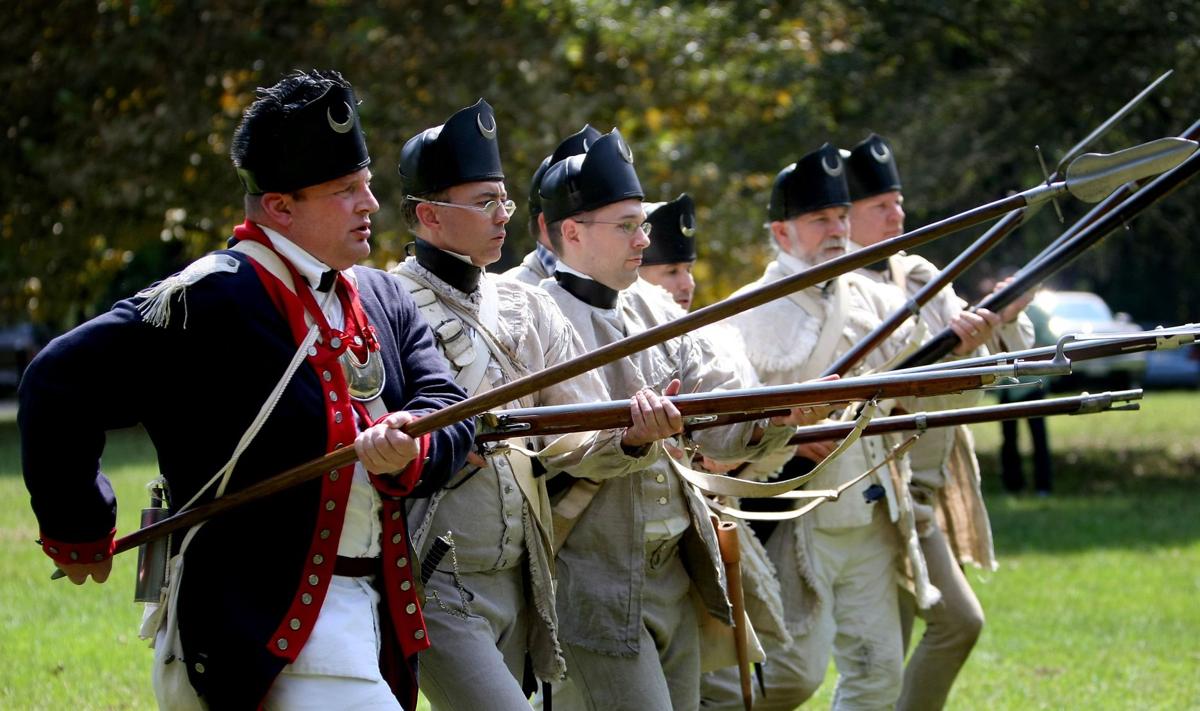The photograph captures a vibrant outdoor scene set in a park with lush green grass and a background of parked vehicles and tall trees. It is evident that the image was taken during the daytime, as sunlight illuminates the scene. The focal point comprises seven men dressed in period military uniforms suggestive of British influence, possibly depicting Minutemen from the Civil War era.

At the forefront stands a distinguished figure, likely the leader, adorned in a dark blue military coat with striking red borders and silver buttons, complemented by a white shirt, white pants, and a black cap featuring a silver crescent-like emblem. He holds a large gold pendant on a red rope around his neck and grips a long spear, pointing it to the right. This figure is flanked by two men dressed in cream-colored jackets and grey pants, and four more in varied uniforms; the two in the background appear less distinct.

Details such as fringed blue uniforms, some cream attire, black hats, and brown long-barrel rifles held by several men enrich the authenticity of this scene, embodying a historical reenactment. The composition, rich in its photographic realism, effectively captures the essence of a meticulously staged historical event amidst the serenity of a park landscape.